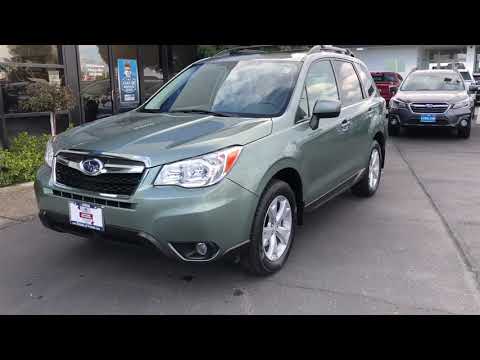The image showcases a relatively new, dark green SUV with a boxy front and curved back, parked on a cement parking lot. Positioned to the side and facing us at an angle, the vehicle appears to be on a car lot, suggested by the presence of several cars behind it that also lack license plate numbers. The SUV has a somewhat blurry insignia, likely a Nissan, and a front dealer plate with a red box, though the specifics are unclear. It has four doors and is parked next to a building with reflective windows and a blue poster that includes a small, indistinct face. In the background, there are additional cars, including a black SUV, a white car, and a red car, all parked in various directions. The scene includes some green grass visible to the left of the main SUV and is framed by a black rectangle at both the top and bottom of the photo.